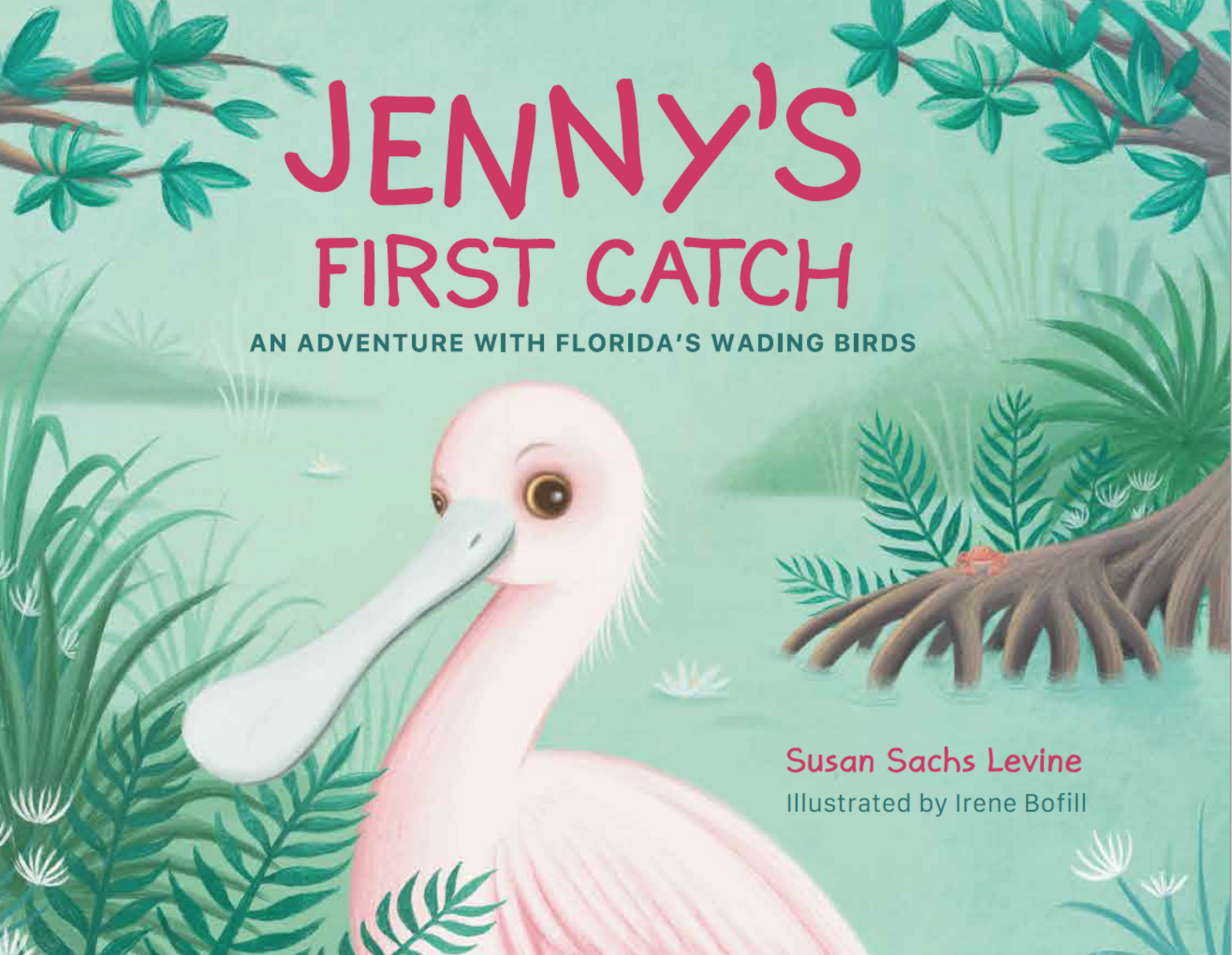The image portrays the cover art of the children's book titled "Jenny's First Catch: An Adventure with Florida's Wading Birds." The title is prominently displayed at the top in red lettering that resembles a child's handwriting, with the subtitle below in a dark blue-green color. Authored by Susan Saxe-Levine and illustrated by Irene Beaufille, their names are respectively written in red and blue-green at the lower right of the cover.

Dominating the lower half of the illustration is a white bird with soft pink shading, likely a roseate spoonbill. The bird faces the left, with a long, broad, flat bill colored gray. Its yellow-rimmed black pupils and light gray eyebrows give it a distinctive look. It stands in a Florida swamp or Everglades setting, surrounded by simplistic ferns, trees, and water. Among the details, there's a pond flanked by green land and a tree with roots stretching into the water, hosting a small orange crab. The backdrop includes painted elements of branches and foliage, creating an authentic Floridian swampland ambiance.